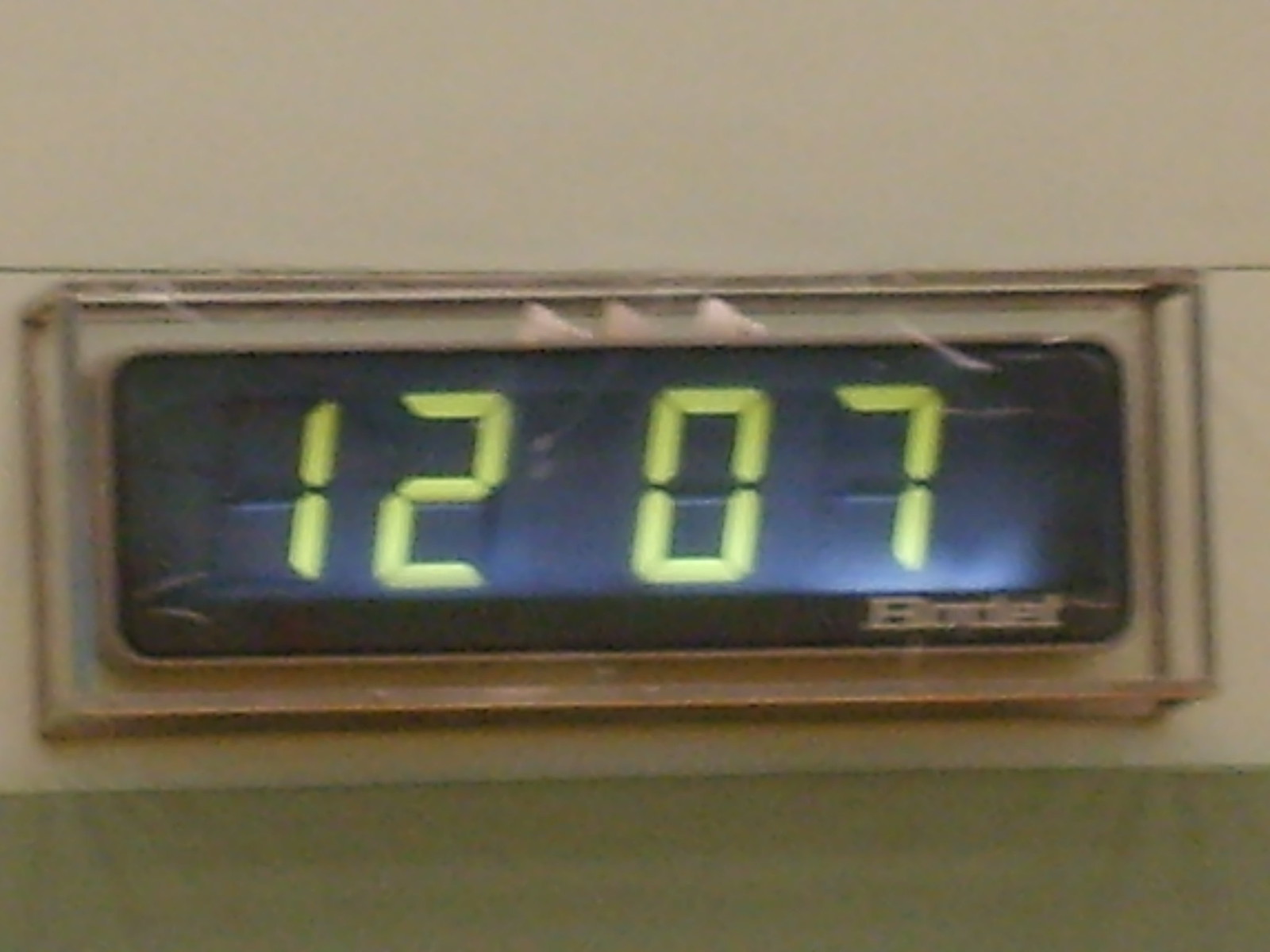The image prominently features a sleek, rectangular digital clock with a black face displaying large, yellow numbers reading "12:07." The clock is framed by a slim, tan-colored trim, which appears to be made of metal, adding a touch of modern elegance to its design. The digital face contrasts sharply with the frame, making the time easily readable. At the bottom right of the clock face, there is a brand name that starts with the letter "B," though the remaining letters are hard to discern. The background of the image is divided, with the upper three-quarters being a warm tan hue and the bottom portion featuring a solid green color that spans the entire width of the frame. The overall composition is minimalistic yet striking, highlighting the clock's contemporary aesthetic.